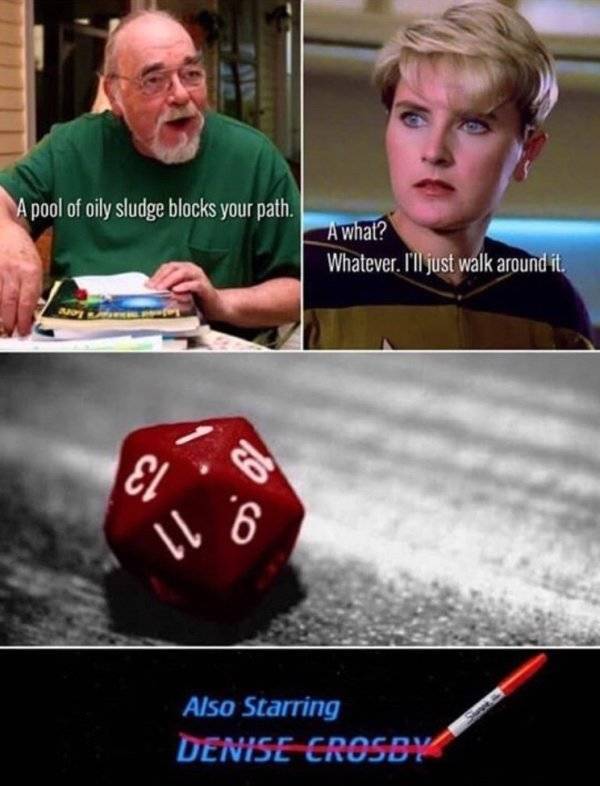The image is a detailed collage divided into four sections, resembling scenes from a movie. In the top-left section, an elderly man with a white beard, wearing glasses and a green shirt, sits in front of a pile of books and papers. He is talking to someone, and the text in front of him reads, "A pool of oily sludge blocks your path." To his right, in the top-right section, a blonde woman in a black shirt with tan and brown accents listens, responding with, "A what? Whatever. I'll just walk around it." 

The bottom-left section shows a colorful, multi-sided dice featuring numbers like 1, 6, 11, 13, and 19. Below this, in the bottom-right section, a black rectangle with blue text reads, "Also starring Denise Crosby." This text is crossed out with a red Sharpie, which is also visible in the frame. The overall style of the image mimics a film scene, adding a narrative feel to the composition.